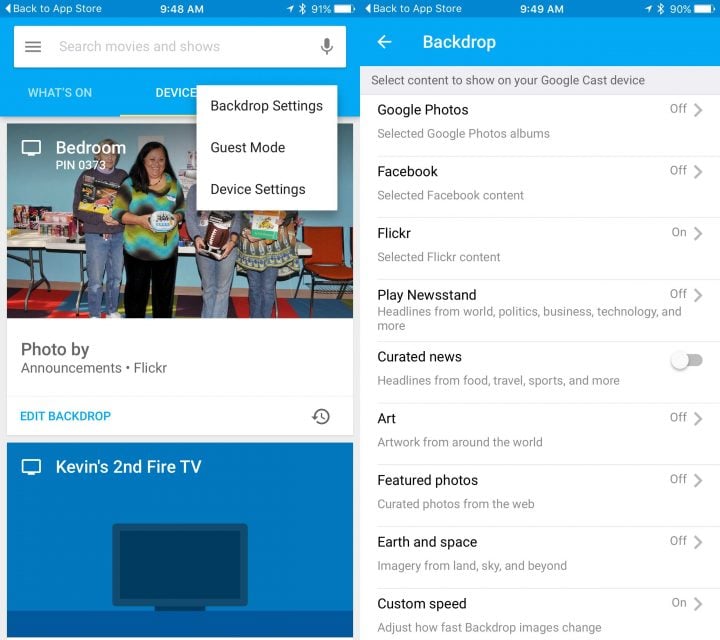This screenshot, likely taken from a mobile device, showcases a blue and white interface for an app that seems to manage display settings for a second Fire TV device named "Kevin's Second Fire TV." At the top of the screen, there is a search bar. Below it, a partially obscured image of four people, attributed to "announcements.flickr," is visible. The obscuration is caused by an open drop-down menu that includes options such as "Backdrop Settings," "Guest Mode," and "Device Settings." Towards the bottom left of the screenshot, an image of a TV set against a blue background prominently features the label "Kevin's Second Fire TV." On the right-hand side of the screen, there's a list for selecting content to show on a Google Cast device, with options including Google Photos, Facebook, Flickr, Play Newsstand, Curated News, Art, Featured Photos, and Earth and Space, each of which can be toggled on or off. At the very top, the interface indicates a timestamp of 9:48 AM and 9:49 AM, a battery life of 91% and 90%, and a back navigation option to the App Store twice, suggesting the screenshot includes elements of a mobile operating system’s status bar.